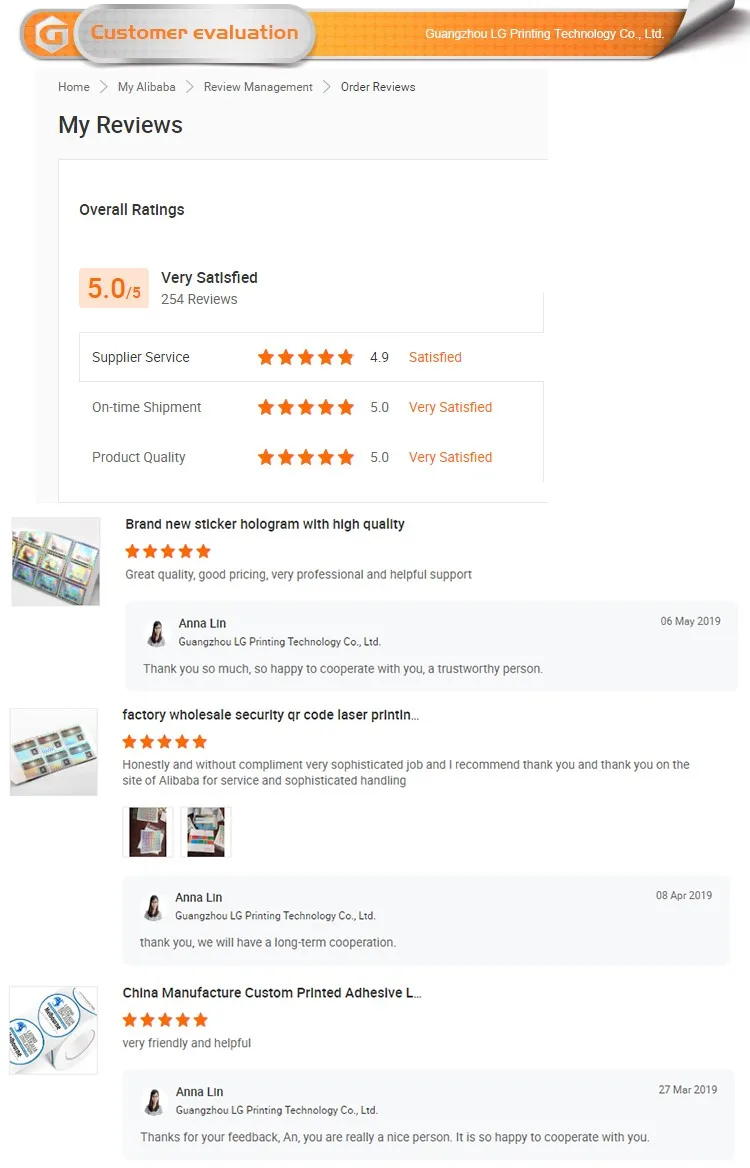The image showcases a section of a website dedicated to customer evaluations of a product. At the top, there's a sleek, grey rounded rectangle featuring a subtle light grey outline and a gradient background transitioning from yellow to orange. On the far left of this rectangle is a silver hexagon with a stylized "G" embossed on it. To its right, overlaid on the first rectangle, is a white rounded rectangle bearing the orange text "Customer Evaluation." Continuously to the right on the first rectangle, which shifts to an orange background, reads the text in white: "Guanzhuzhu LG Printing Technology Co Ltd." A portion of this rectangle also appears to be slightly lifted, casting a shadow beneath it.

Below this primary section is a tiny text trail, indicating the user's navigation path: "Home > My Alibaba > Review Management > Order Reviews." Following this, in bold black text, the heading "My Reviews" is displayed. The next section, contained within a white rectangle, starts with an orange rating "5.0 out of 5," accompanied by the text "Very Satisfied," reflecting "254 Reviews." Below this, another breakdown includes stars and ratings: "Supplier Service: 4.9 (5 stars), Satisfied," "On-Time Shipment: 5.0 (5 stars), Very Satisfied," and "Product Quality: 5.0 (5 stars), Very Satisfied."

Beneath these ratings are three customer reviews, each awarding 5 stars and including images of what appear to be cards. Each review is accompanied by a response from the product seller.